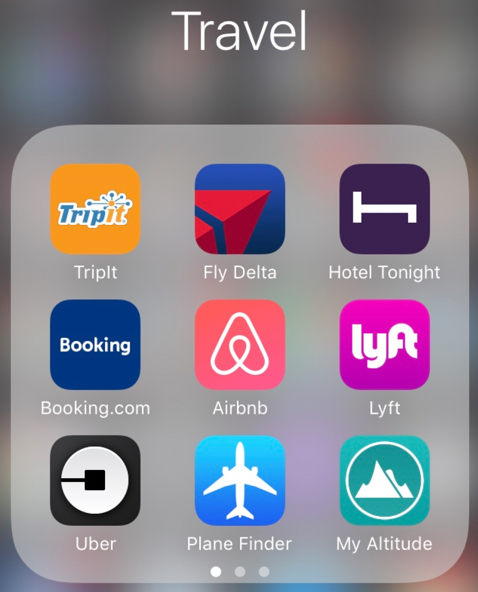This screenshot falls under the heading of "Travel" and showcases nine different apps. From left to right, top to bottom, the apps are as follows:

1. **TripIt**: The app icon features a yellow background with "Trip" written in blue letters and "it" in yellow. Above the text, there is a graphic resembling helicopter blades.
2. **Fly Delta**: This app's icon is primarily blue, featuring a small red triangle intersected by a blue stripe. Another section of red sits in the lower left corner, showcasing Delta's recognizable logo.
3. **Hotel Tonight**: The app icon is dark blue with a simple white outline of a bed symbolizing its focus on last-minute hotel bookings.
4. **Booking.com**: A blue square icon displaying the word "Booking" in white letters.
5. **Airbnb**: This app is represented by a pink square featuring a unique, loopy "A" character.
6. **Lyft**: A neon pink square that contains the word "Lyft" in funky, white letters.
7. **Uber**: A minimalist black square icon with a white circle and another smaller black square inside it.
8. **Plane Finder**: This app's icon is a blue square featuring a white airplane graphic.
9. **My Altitude**: The icon contains a green background with a white circle surrounding a set of mountain peaks.

Each app represents various aspects of travel, from flight bookings and accommodations to ride-sharing and navigational tools.